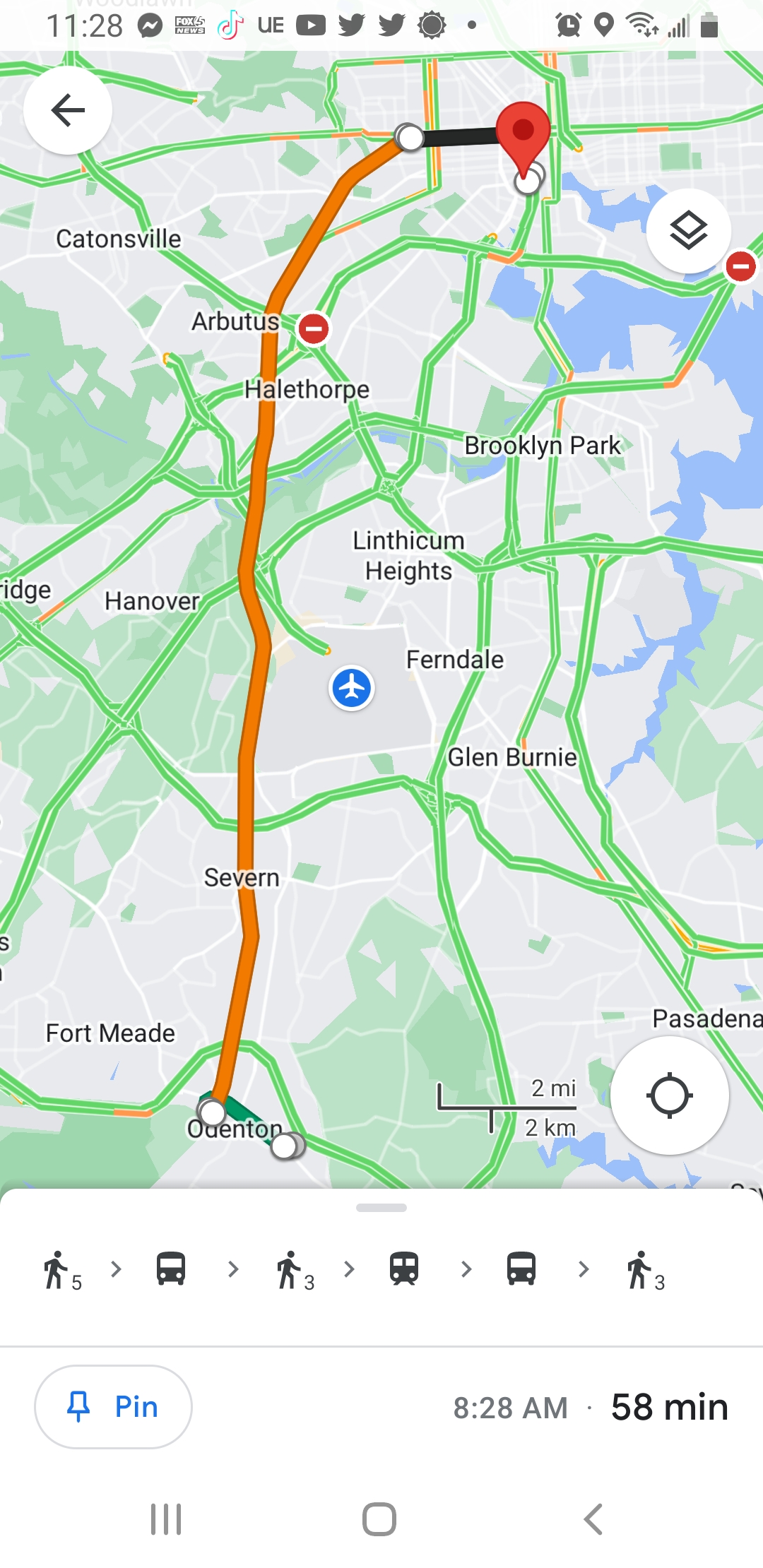The image is a detailed digital map displayed on an Android phone screen, featuring a vibrant design in shades of red, green, gray, white, light blue, and orange. The map shows several geographic locations marked with their names in black text, hovering over their respective positions. Key locations such as Fort Meade, Odenton, Glen Burnie, Ferndale, Linthicum Heights, and Brooklyn Park are clearly labeled. The map includes irregular green lines representing roadways and a highlighted orange line indicating a specific route. This route begins at a dark red arrow in the upper right-hand corner, extending through a black bar and continuing as an orange path towards a destination near Brooklyn Park.

In the lower portion of the map, there are several dark gray or black icons on a white background, accompanied by a blue pin-shaped icon labeled "pin." Just above the bottom are additional details in gray and black text that mention 58 minutes and "8:20 a.m. 5.8 men."

The map is a screenshot taken at 11:28 a.m. on an Android device, as indicated by the phone's status bar showing a 75% battery level, an alarm notification, active location services, and several app notifications including Facebook, TikTok, YouTube, Twitter, and Wever. The bottom of the screenshot features Android's navigation bar with the hamburger menu, home button, and back arrow. The information bar on the map indicates the estimated travel time of 58 minutes with options for walking, bus, and driving, suggesting the person is planning a route to a destination around Brooklyn Park using Google Maps.